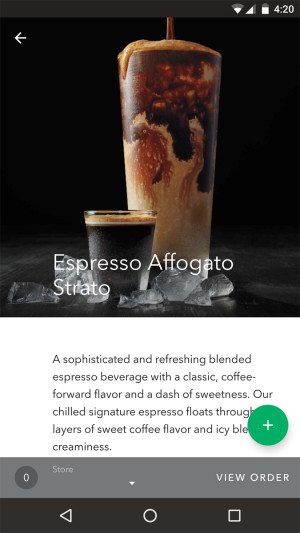This is a detailed screenshot of what appears to be a Starbucks order page. At the top of the page, the time is displayed as 4:20, accompanied by various icons, likely indicating battery level and other device statuses. The main text on the page reads "Espresso Affogato Strato," followed by a detailed description: "A sophisticated, refreshing blended espresso beverage with a classic coffee-forward flavor and a dash of sweetness. Our chilled signature espresso floats through layers of sweet cream, coffee flavor, and icy blend creaminess." There is also a "View Order" button, suggesting that this is a menu or order interface.

In the photograph, the drink is presented in a tall, clear glass with a brown straw. The beverage itself displays a gradient of dark brown and light brown tones, topped with a layer of ice. The table on which it rests is black, accentuating the contrast of the drink. In front of this tall glass sits a shot of espresso in a clear shot glass, characterized by its dark brown liquid and a light brown foam on top. The overall setting evokes a sense of modern elegance, perfect for showcasing this intricately crafted espresso beverage.